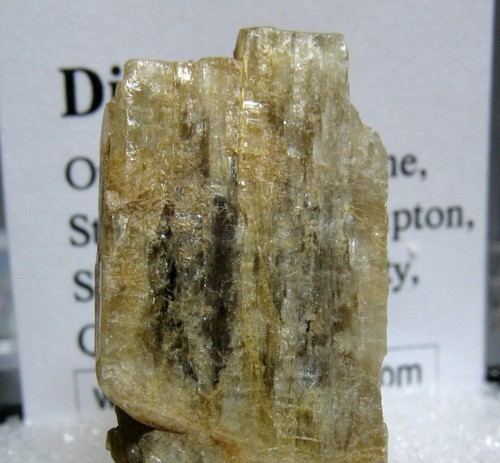This detailed photograph captures a pale yellow rock, possibly jade or another mineral, characterized by dark gray and black streaks, resting on a table indoors. The rock has a vertical rectangular shape with jagged edges and a shiny, crystal-like appearance, reminiscent of quartz. Behind the rock, a white poster with black lettering—partially obscured by the stone—contains rows of text starting with letters such as "D I O S S" and also includes "P H H E, P O N P T O N, Y, N O M" along with the letter "W" visible to the left of the stone. The rock, centered in the image, obscures much of the background document meant to describe the mineral, contributing to the photograph's intriguing composition.